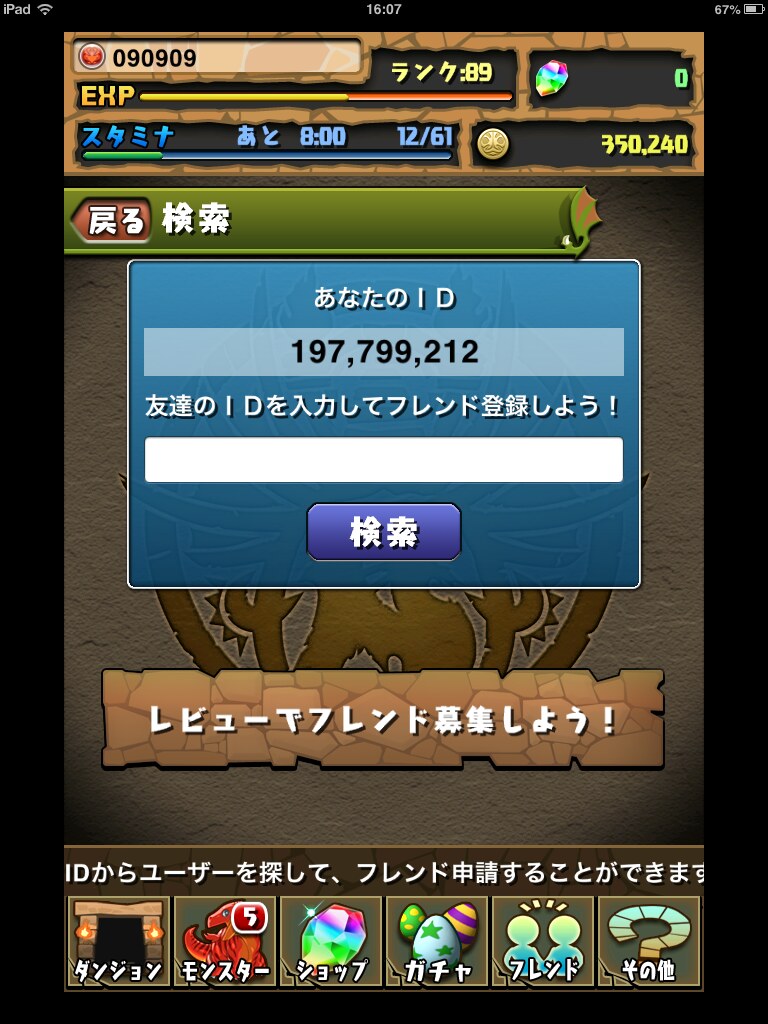This is a detailed color screenshot of a mobile game being played on an iPad, indicated by the text "iPad" in the upper left corner along with a Wi-Fi icon. The time reads 1607 in the middle of the top bar, and the battery indicator on the right shows 67%. The game features an animated interface with text predominantly in Chinese, though some descriptions mention the possibility of Japanese characters. The top of the screen has a series of status bars showing various in-game metrics, including a money counter displaying 350,000 in yellow text. Central to the screenshot is a prominent blue pop-up box featuring an ID number (197-799-212) and other unreadable text in white. The background of the game screen features darker, earthy tones with additional green and blue banners containing more information in both yellow and blue text. At the bottom of the screen, there are six distinct icons representing different game items: colorful Easter eggs with various designs, a multicolored gemstone, a red monster, a cave entrance, and placeholder silhouette icons for additional actions. Overall, the image captures a moment of gameplay with a complex interface rich in visual details and foreign text.